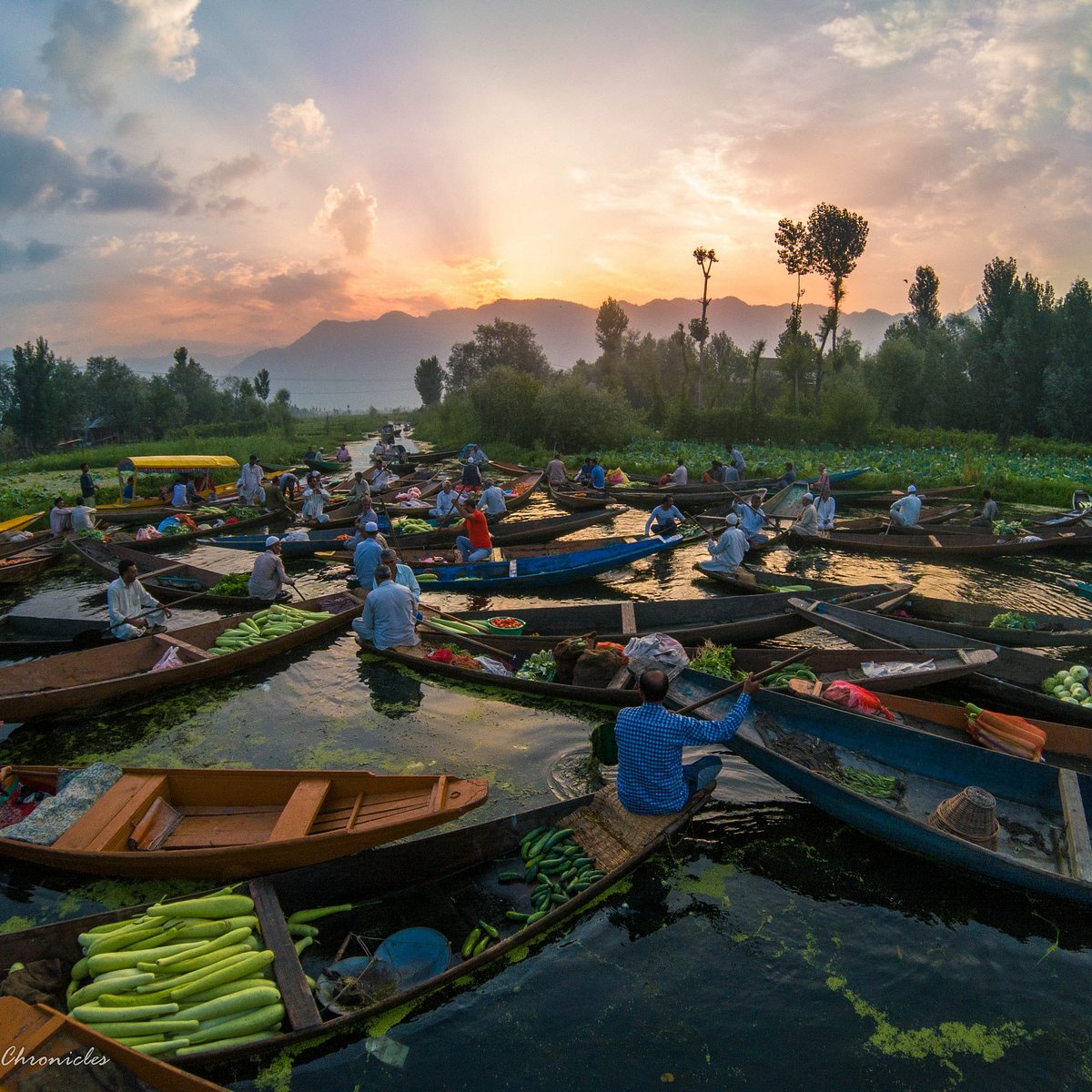In this captivating image, the background showcases a stunning natural landscape at dusk. The sky is painted in soft hues of light purple, orange, and gold as the sun is just about to set, casting a warm glow over the scene. Dominating the horizon is a majestic mountain partially enveloped by a dense array of trees, creating a serene, almost ethereal atmosphere. In the foreground, a tranquil body of water, possibly a river or lake, serves as the setting for the daily activities taking place.

The waterway is dotted with numerous small boats, each manned by individuals who appear to be of Chinese descent. These boats are brimming with large, green vegetables, possibly leeks, which are long and slender, filling the vessels to the brim. The boats are carefully navigating the water as they prepare to unload their abundant harvest. The overall scene is a beautiful blend of nature’s splendor and human industriousness, detailed meticulously with attention to the various elements that together form a picturesque and culturally rich moment.